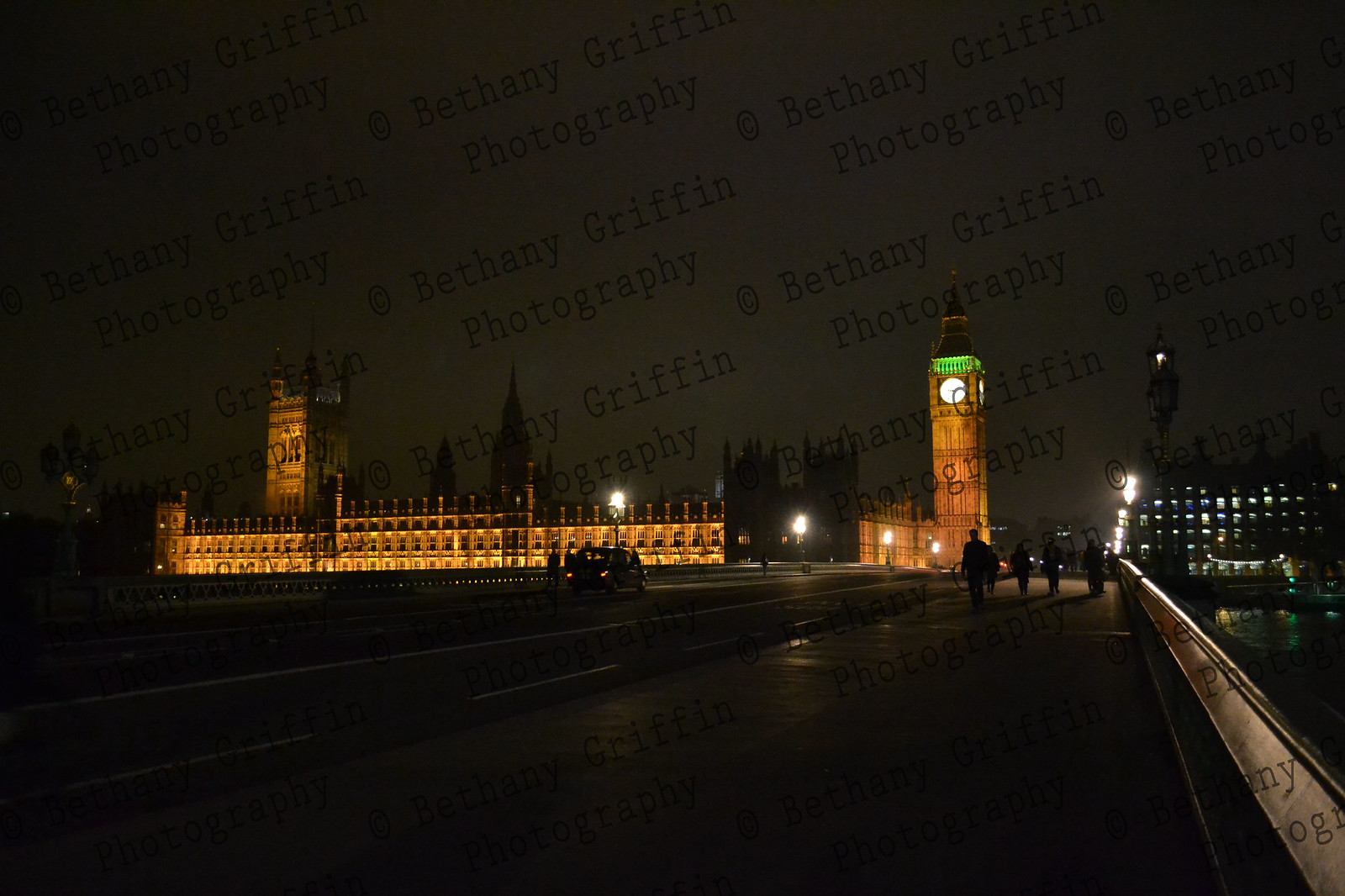This captivating nighttime photograph showcases the iconic Big Ben and the Palace of Westminster, brilliantly illuminated and standing out against the darker surroundings. In the foreground, a sidewalk stretches along with a road, where distant figures can be seen walking and a car is visible further down the street. The majestic Palace of Westminster, a long rectangular structure with an emerging tower, is bathed in a warm golden light, highlighting its intricate architectural details. Big Ben, the tall clock tower with its famous clock face and spire-shaped apex, dominates the middle of the image, exuding an aura of history and grandeur. Superimposed on the image is the text "© Bethany Griffin Photography," marking the composition as a creation of the noted photographer.